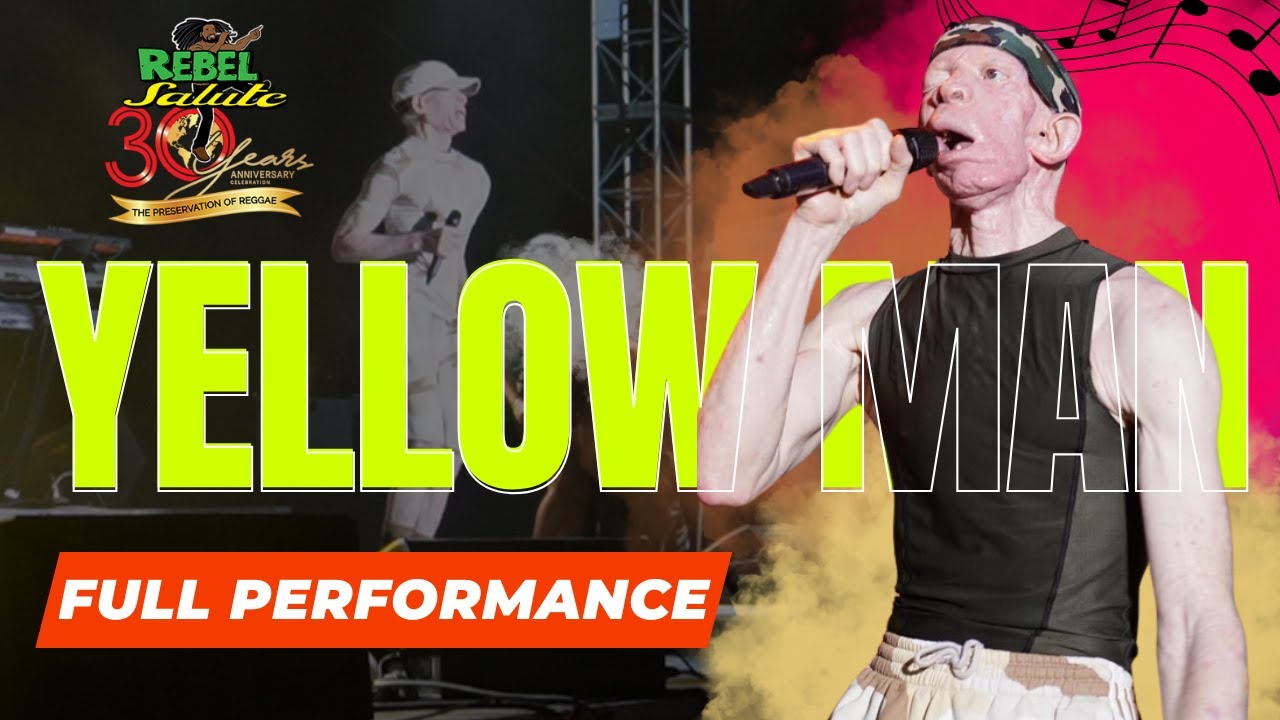The flyer is an advertisement for a performance by the reggae artist Yellow Man. In the center of the image, Yellow Man is prominently featured wearing light-colored camo sweatpants, a black and gray tank top, and a camo-colored bandana. He is holding a microphone to his mouth, with his right eye closed, indicating that he is in the midst of a performance. His distinctive appearance includes pale skin, characteristic of his albinism.

To the left, there is another black and white photo of Yellow Man performing on stage. Beside him, a vibrant yellow smoke engulfs the background, enhancing the lively atmosphere of the flyer. Musical notes can be faintly seen within the colorful smoke on the right side of the image.

At the top left corner of the flyer, a logo in red, yellow, and green reads, "Rebel Salute 30th Anniversary: The Preservation of Reggae." Across the center, bold yellow text displays "Yellow Man," and underneath, in white text set against a red rectangle, it reads "Full Performance." This flyer visually encapsulates the energy and legacy of Yellow Man's contribution to reggae music.